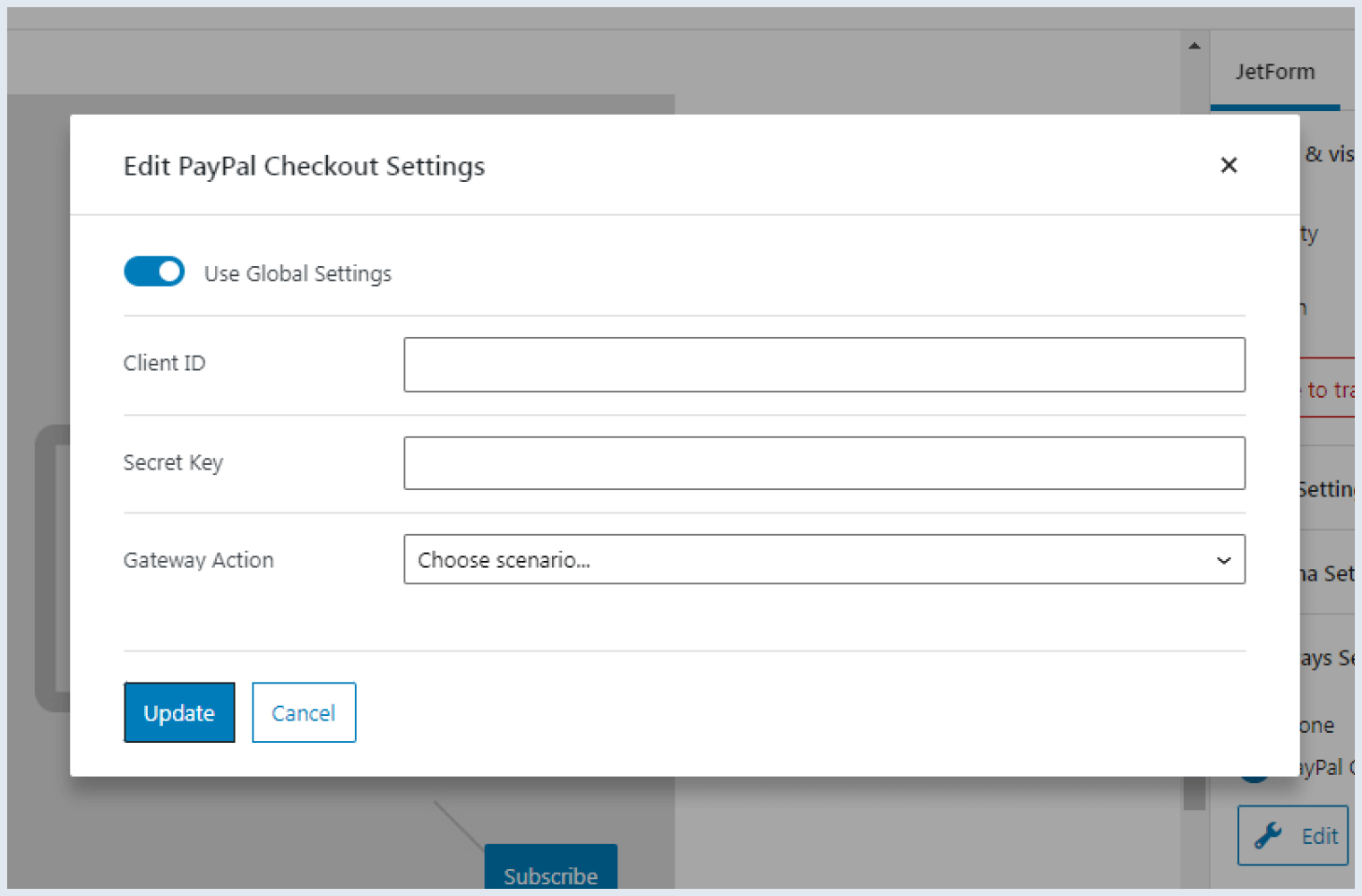The image is a screenshot from a PayPal interface displayed on a desktop or laptop. Dominating the screen is a prominent pop-up window titled "Edit PayPal Checkout Settings" in the largest font. On the left side beneath this title is a blue toggle switch labeled "Use Global Settings," which is currently in the "on" position. The pop-up also includes three labeled input fields: "Client ID," "Secret Key," and "Gateway Action." The "Gateway Action" field is accompanied by a dropdown menu with the prompt "Choose Scenario."

At the bottom of the pop-up, there are two actionable buttons: a blue "Update" button and a white "Cancel" button. The underlying screen, partially obscured by the pop-up, shows a portion of the interface labeled "JetForm" in the upper right-hand corner.